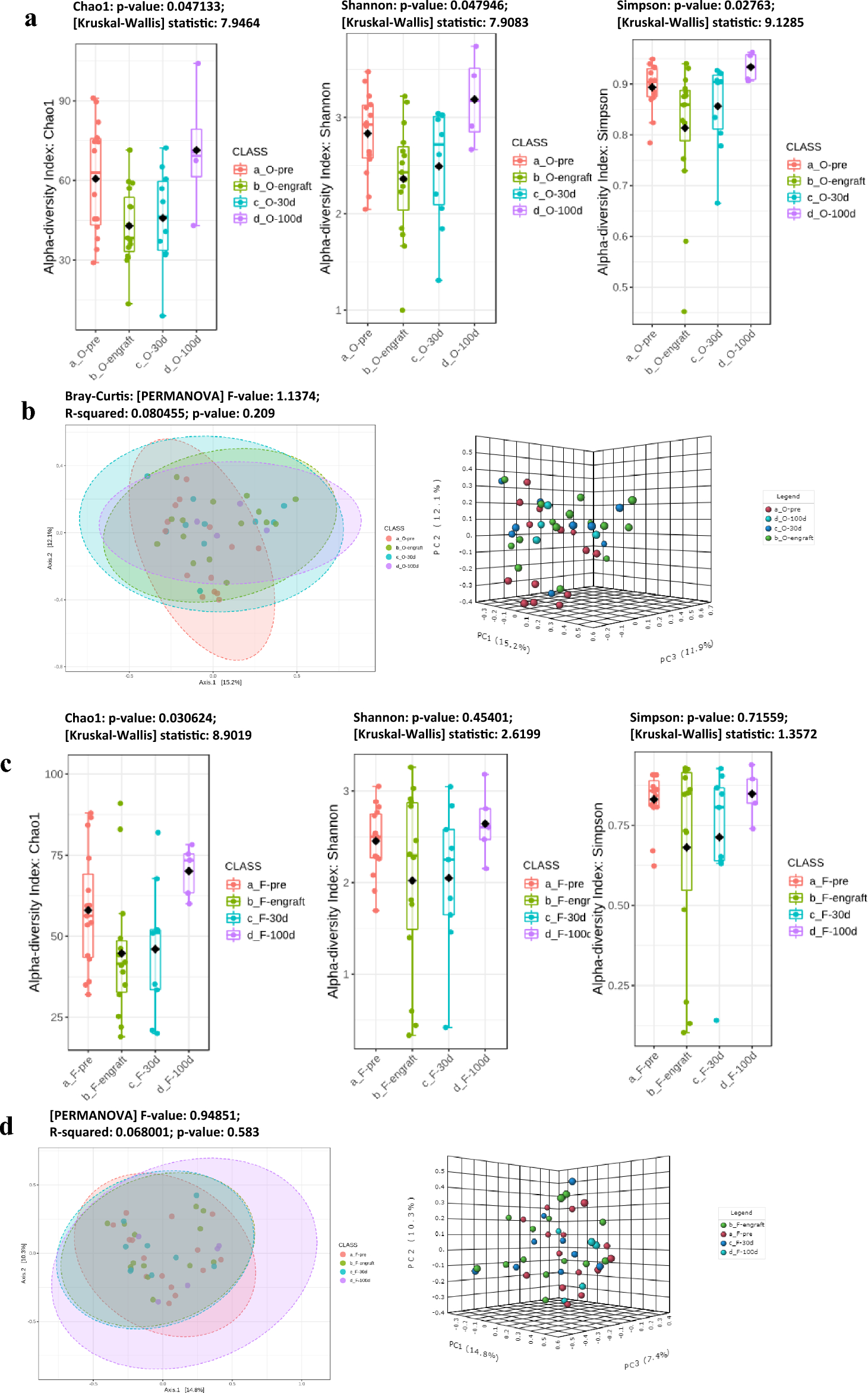The image showcases a detailed poster filled with various scientific diagrams and graphs organized into four labeled sections: A, B, C, and D, against a white background. 

**Section A** features three similar diagrams, each distinguished by colored lines in red, green, blue, and purple, likely representing different statistical data.

**Section B** contains two distinct types of graphs. One showcases overlapping ovals in various colors, probably depicting some categorical relationships, while the other resembles a scatter plot with scattered spheres among small squares, potentially indicating a Bray-Curtis-Permanova analysis.

**Section C** mirrors Section A with another set of three diagrams featuring the same colored lines, maintaining the visual consistency of red, green, blue, and purple.

**Section D**, similar to Section B, includes another overlapping-oval diagram and a scatter plot with colored spheres, showing a repeating pattern in the layout.

Accompanying these diagrams are numerous textual elements that serve to explain the different visual data presentations, although the density of information may render them challenging to read.